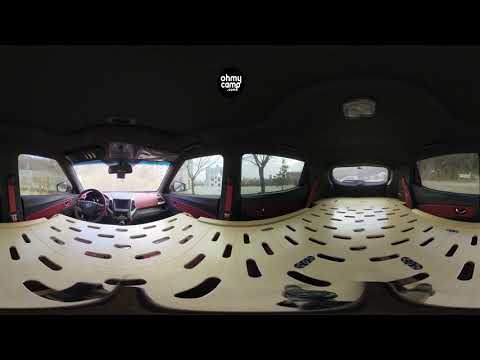The image appears to be taken from inside an unusual vehicle. Dominating the interior is a large piece of white plastic with numerous kidney-shaped cutouts scattered throughout. The vehicle has a black ceiling and red trim around the windows, the steering wheel, and the seat belts. There are six windows spanning the front of the vehicle from left to right. At the top middle of the image, there's a black circular label with white letters that seemingly say "Oh My Camp." The white plastic, with its distinctive cut-outs, seems to cover the floor area instead of the traditional seating arrangement.